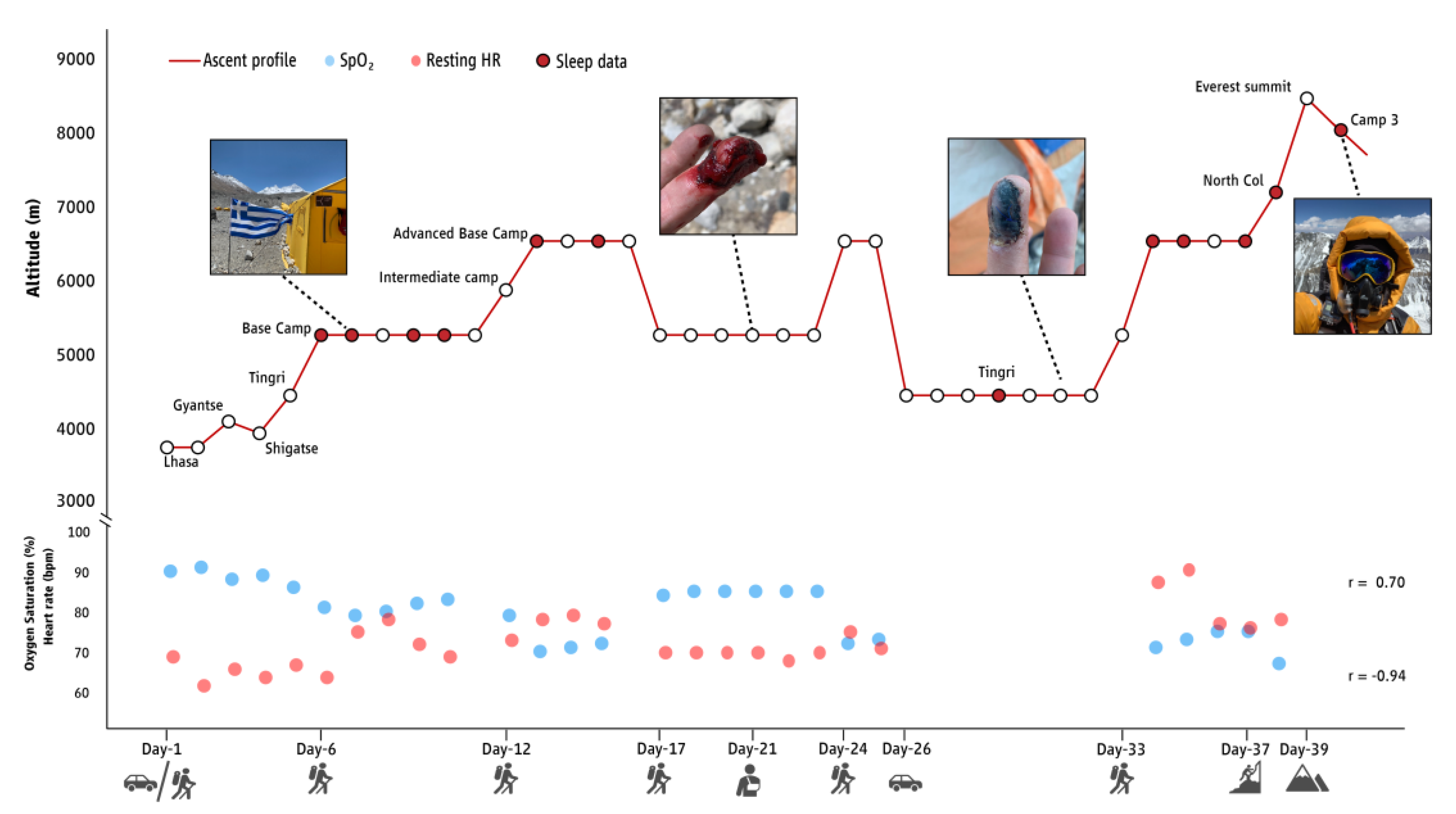This image is a detailed graph charting the progression of an ascent over a period of 39 days. The graph is labeled in black lettering and numbers, with the x-axis showing specific days: Day 1, Day 6, Day 12, Day 17, Day 21, Day 24, Day 26, Day 33, Day 37, and Day 39. Each day is marked with icons; for example, a person walking with a backpack and a stick, a forward slash paired with an automobile, and on Day 21, a figure with an arm in a sling. The last two days feature triangle icons, symbolizing mountains.

Along the y-axis, the graph measures up to 9,000 and includes labels for Oxygen Saturation and Altitude. A key at the top of the graph identifies different markers and lines: a red line for Ascent Profile, a blue circle for SpO2, a pink dot for Resting HR, and a red dot for Sleep Data.

The graph features a scatter plot that spans from the left to the right, with both individual and connected dots forming the data points. Four photographs accompany certain points on the graph, illustrating critical moments: the home base of the climbers, a close-up of bloodied fingers against a rocky background, the same fingers several days later now blackened, and the upper body of a climber in yellow winter gear with a mask and oxygen support system.